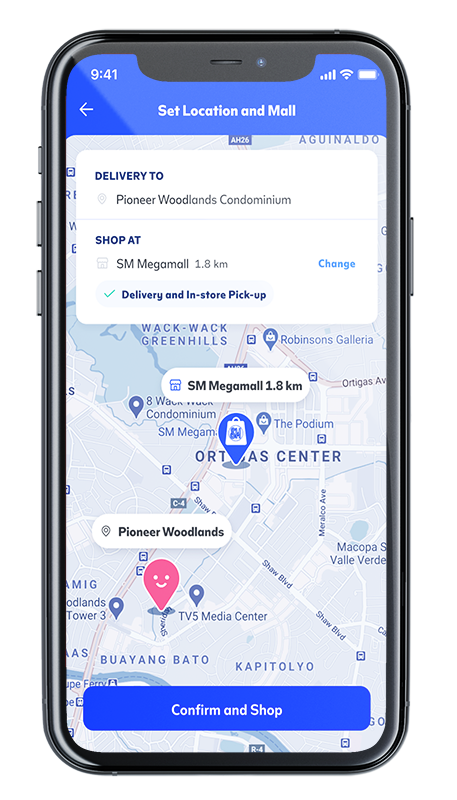**Detailed Caption:**

This screenshot captures the interface of a mobile app designed for shopping or delivery services on a smartphone. The app enables users to set their delivery location and choose a preferred mall for shopping. The interface is well-organized, with several key elements evident:

- **Top Bar:** Displays the current time (9:41) on the left, accompanied by standard signal, Wi-Fi, and battery indicators on the right.
- **Header Section:** Features options to "Set Location" and "Mall, Delivery Location". The user's delivery location is specified as Pioneer Woodlands Condominium.
- **Mall Selection:** Indicates the preferred shopping mall, SM Mega Mall, which is located 1.8 kilometers away. There is a clearly marked option to change the selected mall.
- **Services Offered:** The app provides choices for both delivery and in-store pickup services.
- **Map Section:** Highlights the locations of SM Mega Mall and Pioneer Woodlands Condominium. The map additionally displays landmarks and surrounding areas, such as the Ortigas Center and the Bayayang Bato.
- **Bottom Section:** Features a prominent blue button labeled "Confirm and Shop" designed for user convenience and to proceed with their shopping or delivery.

The app sports a user-friendly design with intuitive labels and icons. The map offers a visual reference for locations, enhancing the overall user experience and making navigation straightforward.